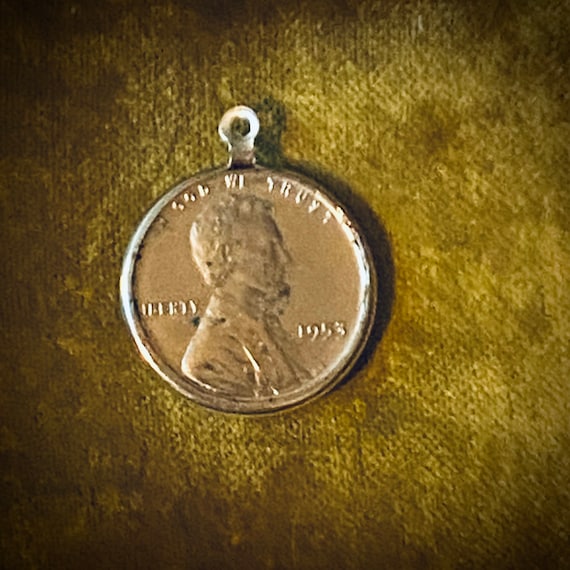The image is a slightly blurry, realistic photograph with a square shape. It features an American penny that has been turned into a pendant, complete with a small loop at the top for attaching to a necklace chain. The penny shows the side profile of Abraham Lincoln, with "In God We Trust" etched at the top, "Liberty" to the left, and the year "1953" on the right. The coin is the regular copper color and appears to be encased in a little metal frame, serving as the medallion part of the necklace.

The pendant rests on a piece of worn, yellowish fabric that resembles burlap or a similar canvas material. This background fabric looks discolored and uneven, with a fuzzy cross-hatching texture that is lighter in the center and darker towards the edges. The overall photograph is dim and slightly blurred, giving it an aged, rustic feel.